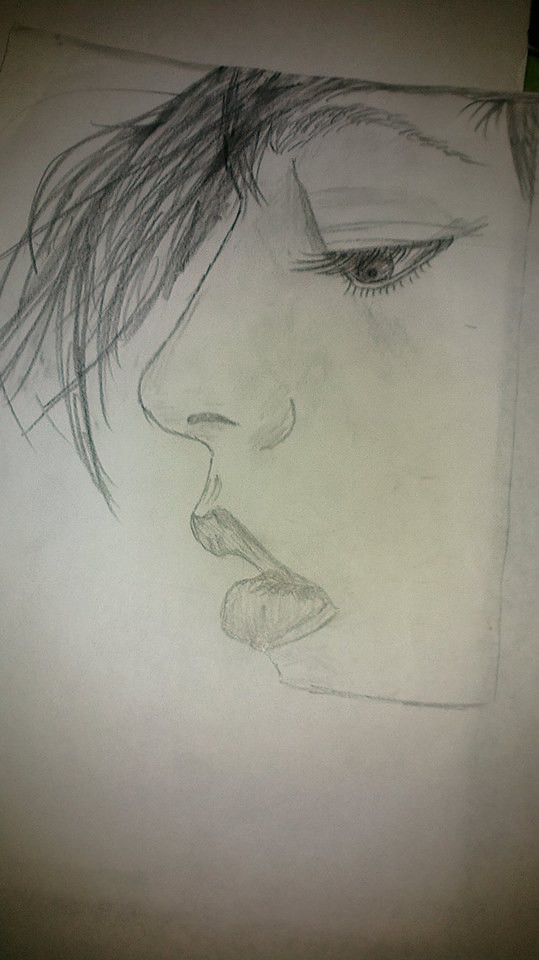The image depicts a detailed pencil sketch of a woman's face on gray or off-white sketch paper. The illustration captures a side profile of the woman, focusing on the left side of her face. She has long black hair that cascades downward and partially obscures her eyes and nose. The woman's eye, complete with prominently sketched eyelashes, is directed downwards. Her eyebrows are finely detailed and her lips, which might suggest the application of lipstick due to the intricacy and darkness of the shading, are slightly parted, revealing subtle lines. The overall shape of the sketch is rectangular, and it is devoid of any text. The gaze and expression of the woman, combined with the meticulous pencil work, convey a nuanced and contemplative mood.